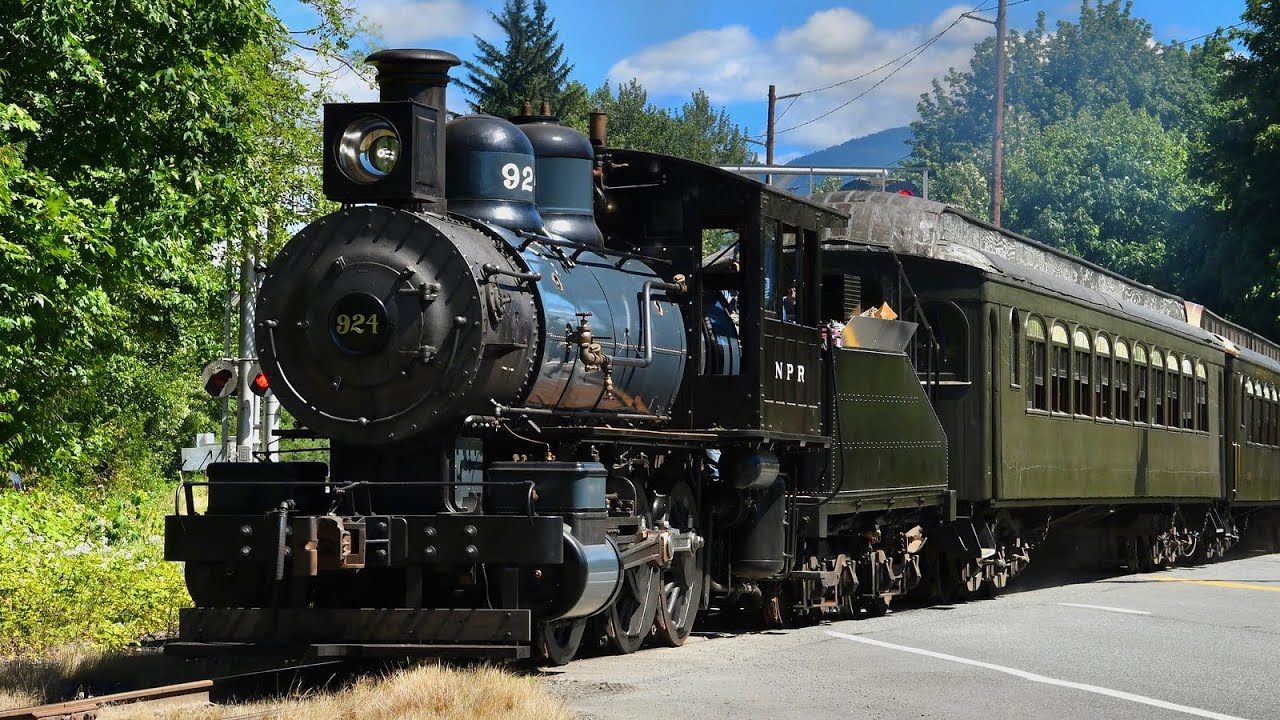This photograph captures an angled view of a vintage passenger train likely displayed for show rather than in operation. The train's black engine car prominently features white writing, including "NPR" at the top and the number "92" across the front. A black circle centered on the front of the engine displays the number "924." The passenger cars trailing behind are a distinct olive green, although the scene does not reveal more than two cars. A blue sky with white puffy clouds and a hint of a mountain peak dominate the background, while trees and grass frame the left side of the image. In the left corner, a parking lot marked with both white and yellow stripes is visible. Additionally, the train’s wheels seem positioned on the track in a peculiar manner, suggesting it's stationary and likely meant for display. A railroad crossing with red lights in the background adds to this impression. The entire scene is accompanied by glimpses of a nearby road and train tracks, contributing to the train's picturesque but non-functional setting.